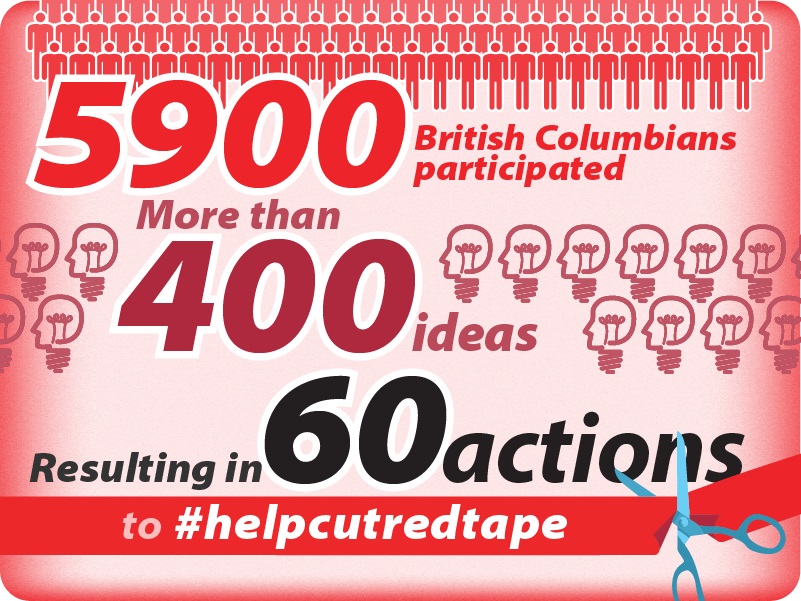This image is a digital poster characterized by its predominantly pink and red rose hues, with accents of black text. At the top of the image, a large group of cartoon-styled people appear in multiple overlapping rows, signifying a crowd. Just below this crowd, text in black reads "5,900 British Columbians participated," followed by "more than 400 ideas." Surrounding the central section, cartoon light bulbs shaped like human faces are dispersed on both the left and right sides, adding a playful touch. At the bottom, the poster declares in text, "resulting in 60 actions to #help cut red tape," emphasizing a social media initiative. The bottom right corner features a blue pair of scissors cutting a ribbon, symbolizing the action of reducing bureaucracy. The background colors include shades of red, pink, white, blue, maroon, and gray, giving the poster a vibrant and engaging appearance.